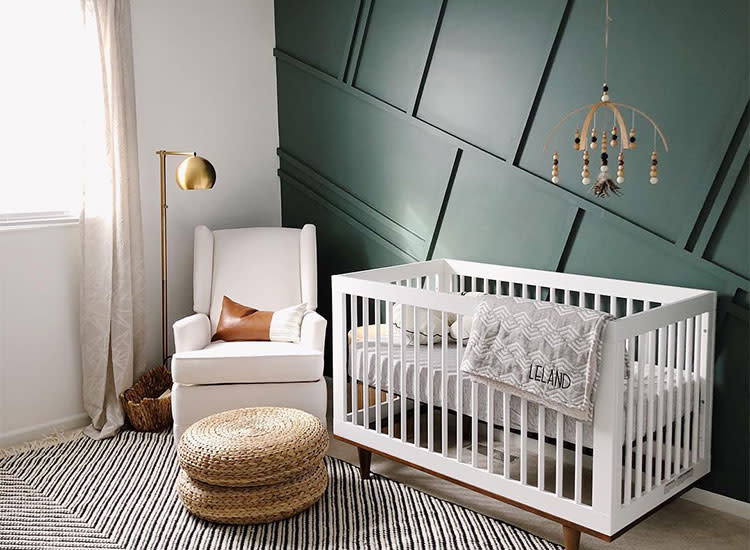The nursery is a beautifully designed space, likely captured by a professional photographer. At the center, a white wooden crib with dark posts is prominently placed against a striking dark green wall, which has a 3D textured and wooden beam detail separating white segments. Over the front rail of the crib hangs a gray blanket with white zigzag patterns, stenciled with the name "Leland" in capital letters. Inside the crib, a cream-colored circular pillow, commonly known as a "boppy," adds to its comfort.

Adjacent to the crib, a cozy sitting area features a white stuffed chair adorned with a brown and white pillow, paired with an interlocking wicker footrest and a matching brown ottoman. The wall beside this setup is white, showcasing a large window dressed in floor-length white shades with beige curtains, allowing ample light to flood the room. A gold lamp sits on a side table near the chair, ideal for nighttime feedings or story time.

Above the crib, a whimsical mobile hangs from the ceiling, decorated with beads and brown and white dots, ready to gently swing and entertain baby Leland. The dark gray striped carpet on the floor ties the elements together, completing the serene and stylish atmosphere of this nursery.